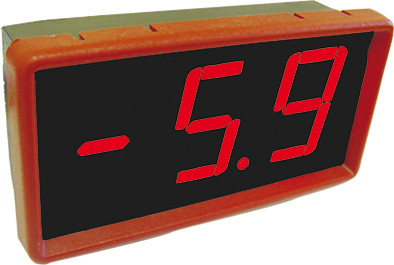The image features an object resembling an alarm clock, set against a plain white background. The device has a predominantly brownish-gray and tan back, with only a small portion visible. Encircling the face of the clock is a fairly thick, reddish-orange rim with subtle grooves at the top. The clock face itself is black, displaying the numbers "5.9" in a digital, segmented style typically associated with alarm clocks.